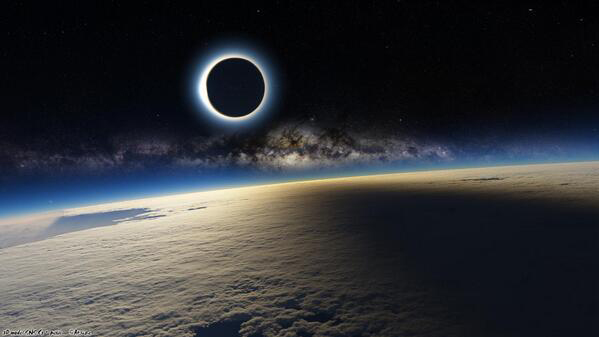The image is a rectangular horizontal photograph, almost twice as wide as it is tall. The scene is set in outer space, capturing a breathtaking view of a solar eclipse. At the center top of the image, we see a large black circle which is likely the Moon, partially obscuring the Sun, creating a glowing white rim around the eclipse that is brighter on the left side. Crowning the scene is a band of black that fades into a deep blue as it transitions downwards, blending with the line of ethereal clouds or possibly nebulae stretching across the frame.

Beneath these clouds, a slightly curved blue expanse represents Earth's atmosphere, arcing upwards to the right. The surface below this layer appears as a cloud or snow-covered planet, showing Earth in mid-eclipse with shadows cast dramatically over its craggy, reflective white terrain. The surface features a shadow in the upper left corner and another steep shadowed incline on the right, creating a striking contrast between light and dark regions.

In the backdrop of the eclipse, the nearly black sky is dotted with faint stars, giving a mild view of our galaxy, the Milky Way. This cosmic tableau is likely from a science magazine, showcasing a carefully composed, scientifically significant moment captured in the last two decades.